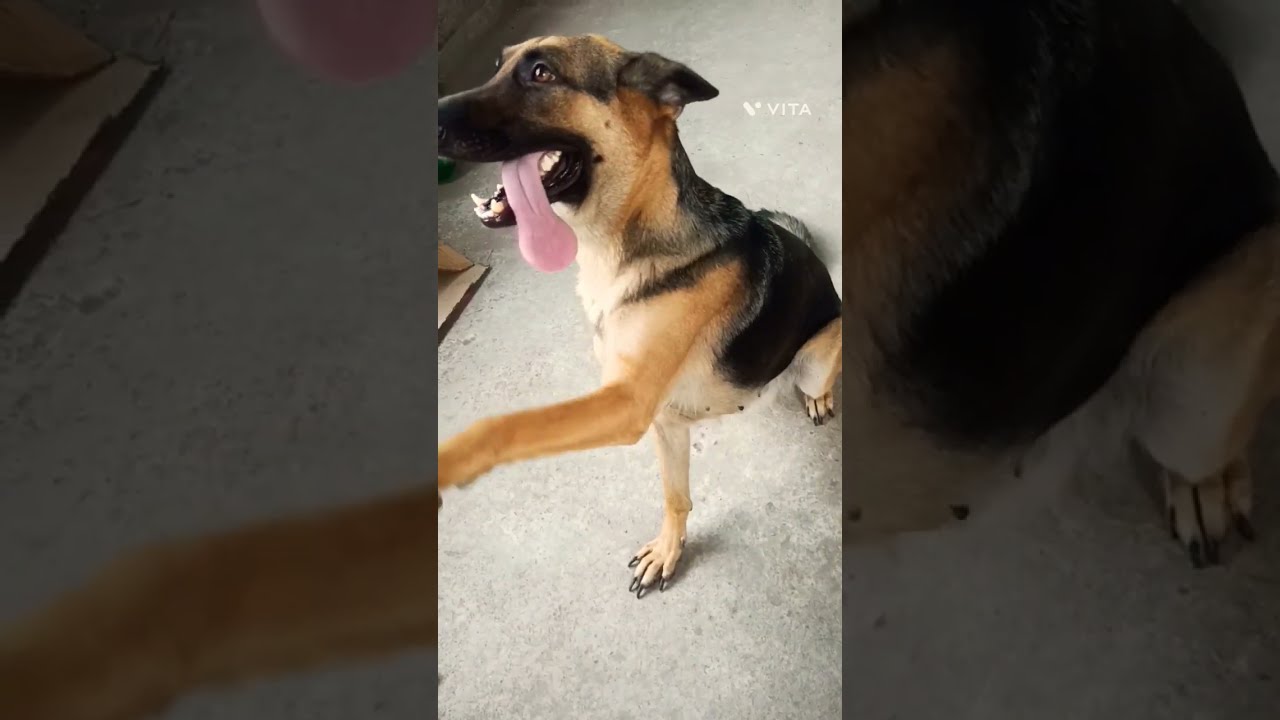The photograph features a German Shepherd mix, potentially with Labrador or Terrier, sitting on a gray concrete floor. The dog exhibits a coat of black, brown, and white, with a black muzzle and back, and brown in between. Its mouth is open, showcasing white teeth and a long pink tongue hanging out to the side. The dog’s left front paw is raised, possibly suggesting a handshake. Notably, it has long black toenails on the grounded paws, in need of trimming. The image is centered with enlarged and darkened repeated sections of the original photo on both the left and right sides. A watermark reading "V Vita" is visible in white at the top right corner.